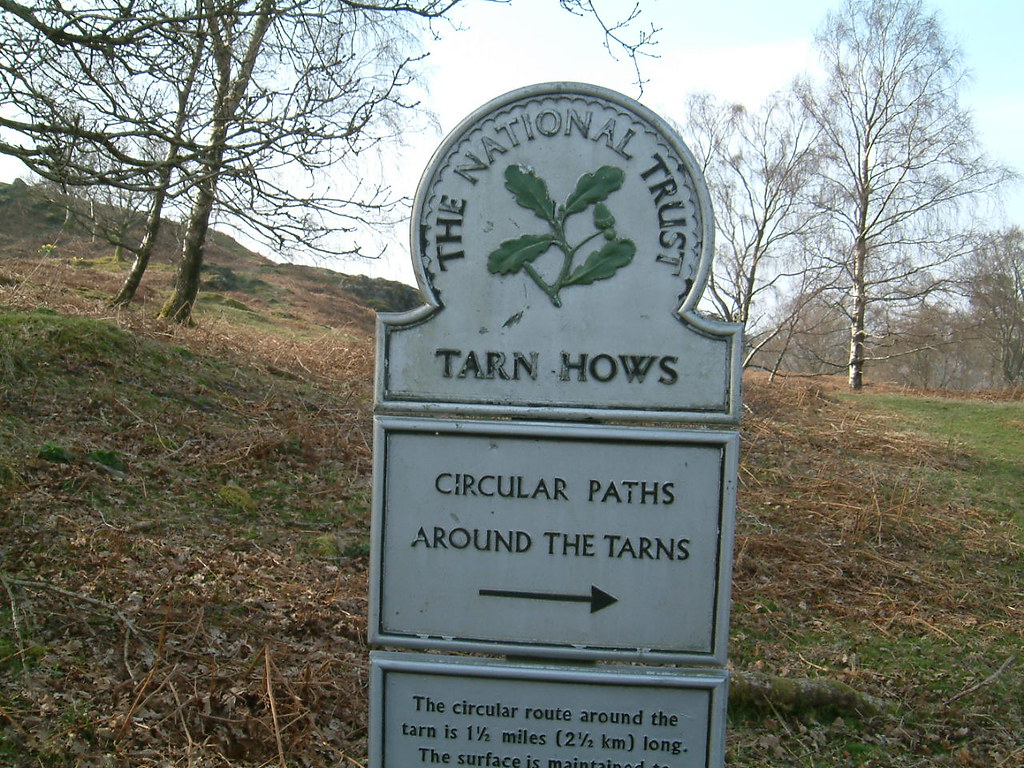The outdoor image features a prominently positioned, white, three-sectioned sign from the National Trust. The top section is circular, displaying the words “The National Trust” around an emblem depicting a green branch with leaves and an acorn. Below this emblem, the words “Tarn Howes” are inscribed. The middle section of the sign provides directional information, stating “Circular paths around the tarns” with an arrow pointing to the right. The partially visible bottom section explains that “The circular route around the tarn is one and a half miles (2.5 kilometers) long.” It also mentions that the surface is maintained, though the remaining text is cut off in the image. The sign is flanked by gently inclining hills with patches of green and brown grass interspersed with sticks. In the distance, sparse, leafless trees allow glimpses of a blue and white sky through their branches. The overall scene suggests a serene, natural setting ideal for a leisurely walk.